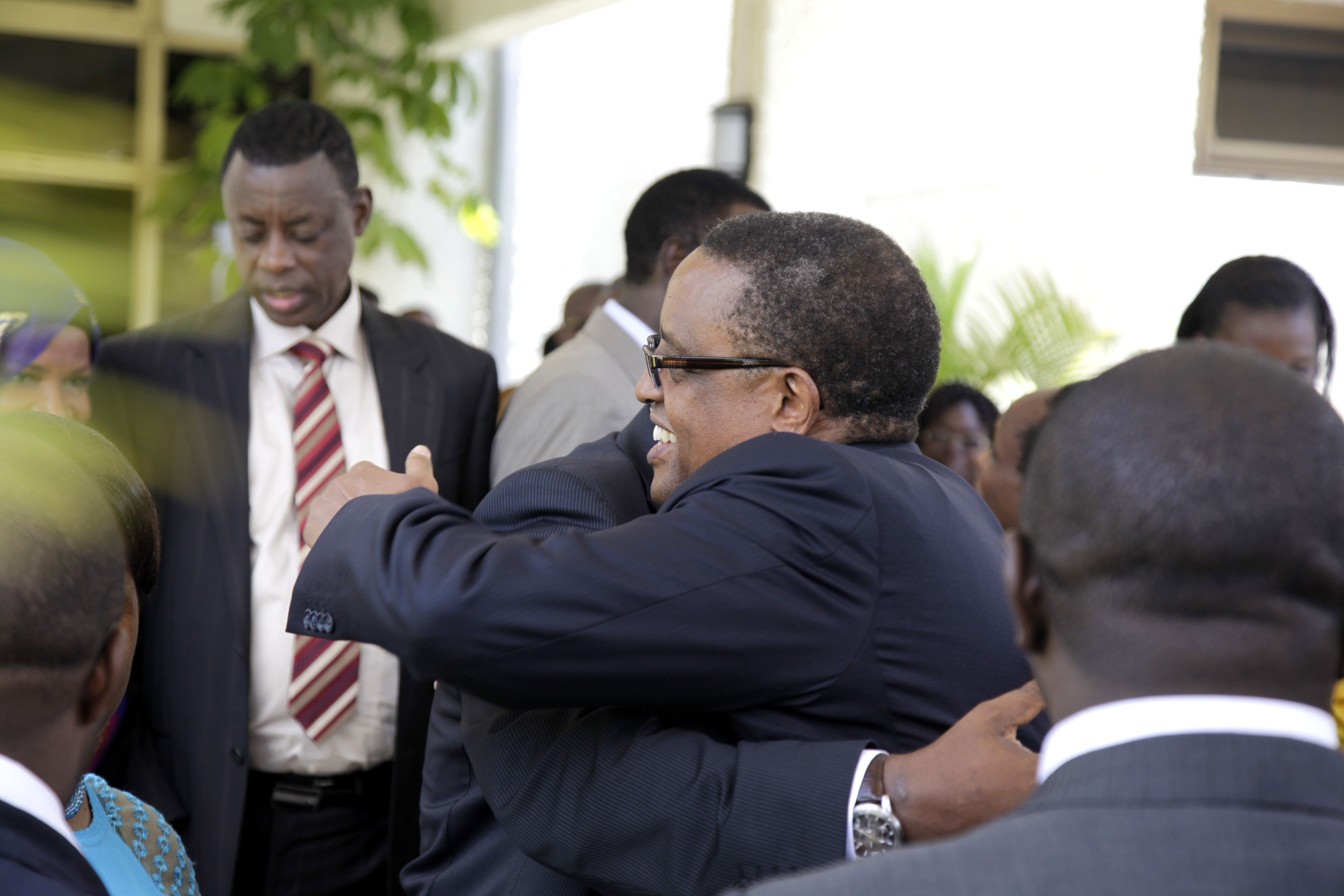In this image, we observe a clear indoor setting likely capturing a moment during an event. The background is a wall that appears mostly plain, with some decorative elements such as plants and shelving visible around it. The main focus of the composition is a group of people positioned directly in the center. Among them, two men are embracing warmly, surrounded by others who are either seated or facing away. The color palette of the scene includes white, tan, brown, black, red, maroon, light blue, and light green, adding a rich diversity to the image. The ambiance suggests a daytime gathering, characterized by a mixture of social interactions and quiet observation.